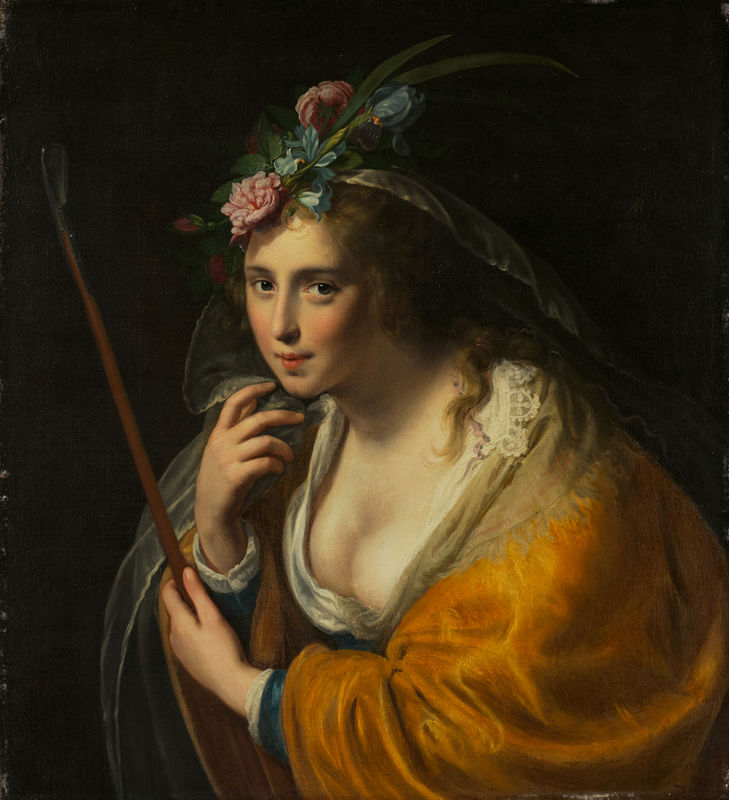This artwork depicts a woman from the 16th or 17th century, illustrated in what appears to be a famous painting set against a stark black background. The woman’s face is angled slightly to the left, revealing her dark brown, wavy hair cascading over her left shoulder and down her back, suggesting it is shoulder-length or longer. Adorning her hair are blue and pink flowers interspersed with vibrant green leaves, which may include dried flowers or feathers. A veil, attached to the floral arrangement, drapes behind her hair.

She wears an elaborate orange-red dress accented with a white-bordered neckline that frames her cleavage, complemented by lace detailing at the neck. Her arms are trimmed in navy blue cuffs with additional lacework. Draped over her shoulders and partly down her right arm is a yellow, gold-colored shawl, enhancing the elegance of her attire.

The woman is full-figured, with fair skin, rosy cheeks, and dark eyes that convey a sly, yet poised expression. Her right hand is raised to her chin while her left hand holds a distinctive staff or wand. This staff, featuring a black wooden handle capped with black metal shaped like a spatula or spoon, suggests a symbol of authority or status.

Her headdress is a lavish combination of floral elements and possibly tulle or chiffon, contributing to her regality. The painting, capturing her from the waist up, vividly illustrates the detailed fashion and intricate accessories of a woman from centuries past, offering a glimpse into the elegance and complexity of historical attire.